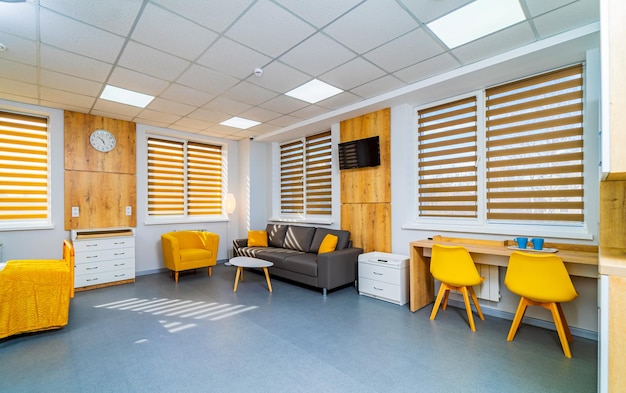This image showcases a well-lit interior scene, likely an office or a school break room, characterized by its modern decor and a clean, minimalistic design. The walls, painted a crisp white, feature seven windows covered with wood slats, interspersed by two wooden panels. One of these panels hosts a clock, possibly alongside outlets or switches, with a white cabinet positioned on the left. 

To the right of the white cabinet is a yellow-armed sofa, situated next to a three-cushioned gray sofa adorned with two yellow accent pillows. A small coffee table stands in front of the gray sofa. Adjacent to this setup is another small cabinet and a desk accompanied by two yellow chairs. The room has a consistent color theme of gray and yellow, adding a cohesive and stylish touch to the decor.

The ceiling is sectioned with four flat lights providing illumination. The flooring is a light gray color, complementing the overall aesthetic. Additionally, there is a very small TV, around 27 inches, mounted on the wall, although it appears impractical for viewing due to its size and positioning. This meticulously arranged space combines function and style, lending it a distinct and orderly ambiance.